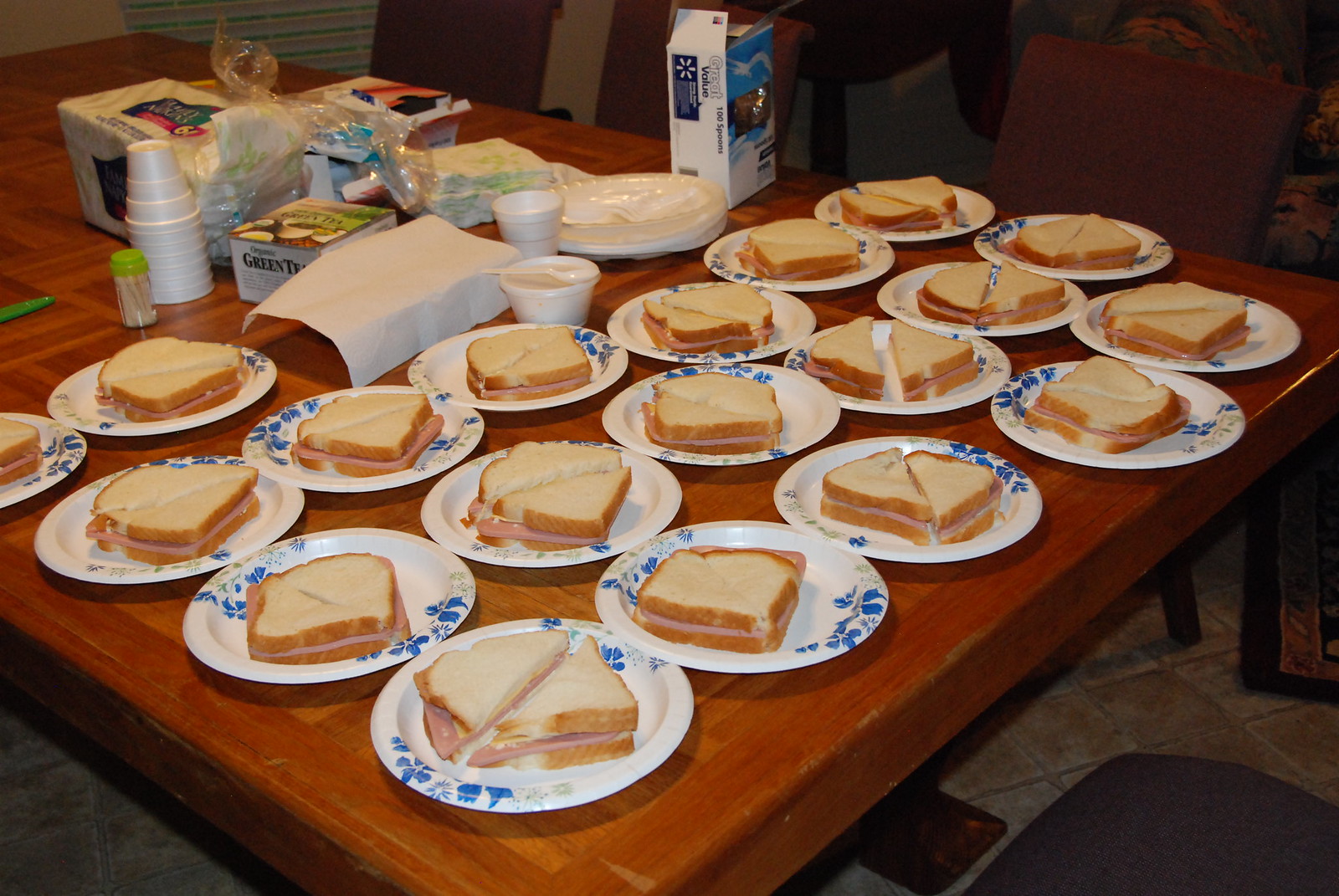In this color photograph taken indoors, we see a rectangular brown wooden table laden with 18 white paper plates, each adorned with a blue floral design. Each plate holds a sandwich made with two slices of slightly toasted white bread, encasing a pale brown meat, likely ham or turkey, topped with yellow cheese. The sandwiches have been neatly cut into triangular halves. The table also features assorted items including a stacked arrangement of white styrofoam cups, a small styrofoam cup with a plastic spoon resting on its lid, a container of toothpicks with a green top, a box of green tea, a blue and white carton of plastic spoons from Great Value, and some napkins. Additionally, the table is accompanied by several brown chairs and a gray chair, completing the setup.